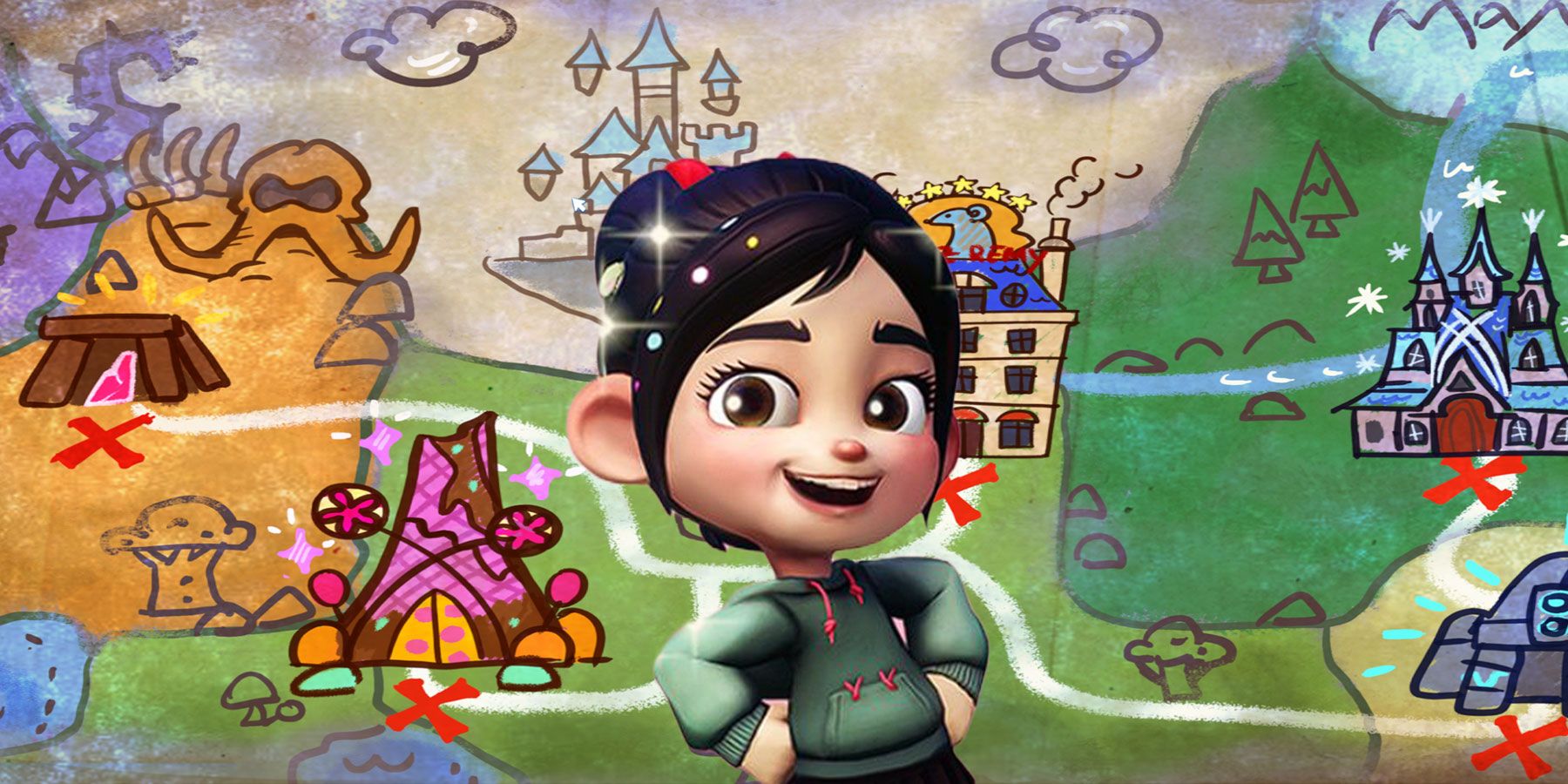This digitally created image features a cartoon-like, young girl who appears to be Vanellope from the movie Wreck-It Ralph. She stands confidently at the forefront of the scene, dressed in a green hooded sweatshirt with red trim and drawstrings, black pants, and a red hair tie securing her black ponytail. Her big brown eyes are full of life as she smiles, her hands firmly placed on her hips.

The vivid and colorful background resembles a whimsical treasure map with fantasy elements. A castle is set against a gray sky tinged with purple hues and dotted with purple clouds. A purple dragon emerges, adding a touch of menace. An angry-looking octopus is also present, enhancing the fantastical atmosphere. A brown bench with a pink gemstone underneath and an 'X' in front suggests a hidden treasure. Moving rightward, the scene transitions into a gentle green hillside adorned with verdant trees and another castle with an 'X' at its entryway. There’s also a tiny house with a mouse perched atop it, further contributing to the rich tapestry of animated elements. The scene is adorned with a variety of colors—purples, greens, blues, and reds—completing this intricate and engaging digital illustration.